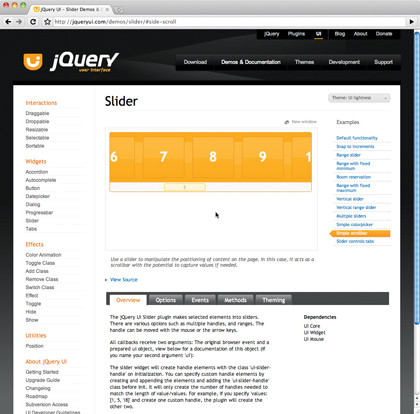The image depicts a web browser displaying the jQuery website. In the upper left-hand corner, the jQuery logo is prominently featured. The logo consists of a lowercase "j" followed by the uppercase letters "QUERY" (Q-U-E-R-Y), accompanied by a yellow, roundish block with a "j" in the middle. 

Located on the upper right-hand side, there is a horizontal top menu with options such as "Download," "Demos," "Documentation," "Themes," "Development," and "Support." 

Beneath this header menu, the main content of the website appears in a large white section. On the left-hand side of this section, a vertical menu lists five different sections. To the right of this vertical menu, a section labeled "Sliders" is visible. This section features a bar, which is segmented and numbered with yellow blocks.